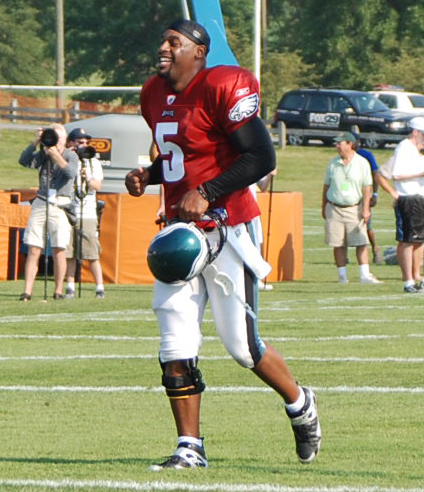The image captures a lively scene at a football training camp, prominently featuring Philadelphia Eagles' player Donovan McNabb. Positioned in the center of the frame, McNabb is seen walking across a football field, holding his helmet in his hand and smiling. He is wearing his team jersey with the number five, white football pants, and a brace below his right knee. In the background to the left, a camera crew with their equipment on monopods can be seen, diligently capturing the action. On the right side of the image, several people stand on the sidelines in shorts with name tags, likely officials, coaches, or media members. Behind them, various cars in colors such as red, light green, yellow, orange, grays, beige, and brown are parked in front of a forested area. One of the cars bears a label with the text "Fox." The setting is clearly on a football field, perhaps during a lively training session.